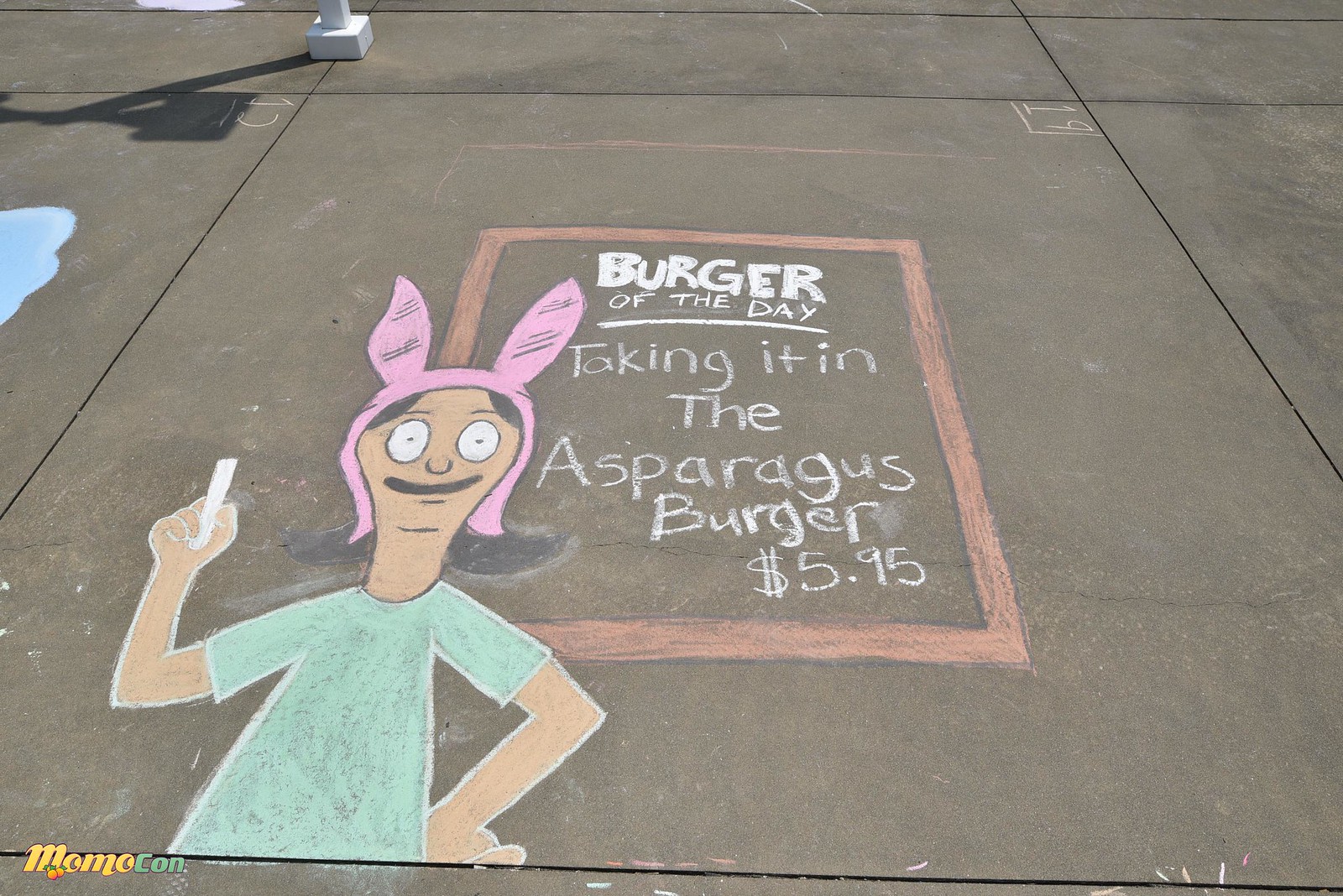This image captures a charming and colorful sidewalk chalk drawing designed as an advertisement. The central character is a cartoon figure from the adult animated show "Bob's Burgers," specifically Louise Belcher, who is known for her iconic pink bunny ears. She is depicted with a big smile on her brown face, white eyes, and is wearing a blue shirt. Louise’s right hand is raised, while her left hand rests on her waist. 

The advertisement itself is skilfully integrated into the drawing. Positioned in the center of the sidewalk, an orange rectangle encompasses the white chalk text: “Burger of the Day,” followed by the special, “Taking It in the Asparagus Burger, $5.95.” This playful design suggests that Louise is presenting the daily special to passersby.

In the lower left corner of the drawing, the signature “Momo Con Dot” is visible, hinting at the artist or the event. Additionally, the upper left corner of the sidewalk shows the base of a white post, and a portion of another chalk drawing is seen on the adjoining part of the sidewalk. Notably, there’s a touch of blue - matching Louise’s shirt - in both the character and the overall layout, adding to the cohesive and enticing visual appeal of the advertisement.